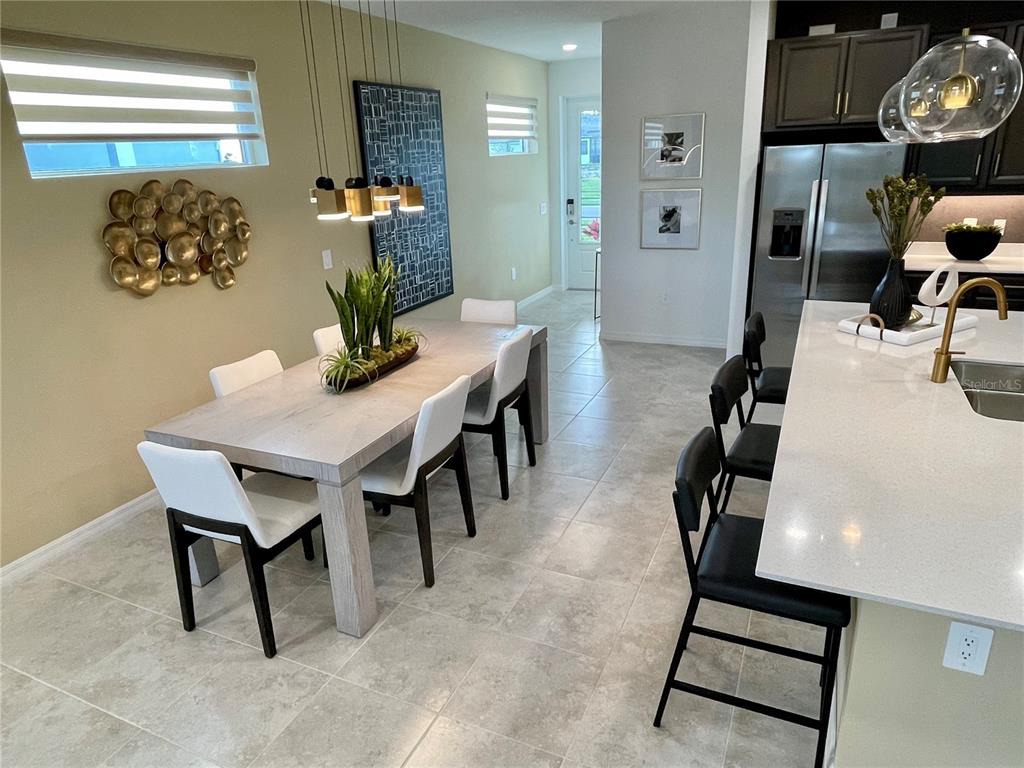This photograph captures a modern, meticulously designed kitchen and dining area. The kitchen features sleek black cabinetry complemented by stainless steel appliances, including a refrigerator. A white marble countertop island is adorned with three black stools, while pendant lights with clear glass globes illuminate the space. Adjacent to the kitchen, the dining room boasts a rectangular hardwood table surrounded by six white chairs with black legs, enhanced by a modern chandelier hanging above. The dining area is accentuated by taupe-colored walls, featuring contemporary artwork—a black-toned painting resembling a stratified brick pattern and two smaller photographs on a divider wall. The wall also displays a bulbous gold statue and a metal sculpture positioned below a window with a shade. Natural light streams in through an additional window and a back door, highlighting the light tan, white, and black palette of the room. The flooring throughout the space appears to be a gray-tiled surface, resembling travertine marble, adding to the room's sophisticated ambiance.